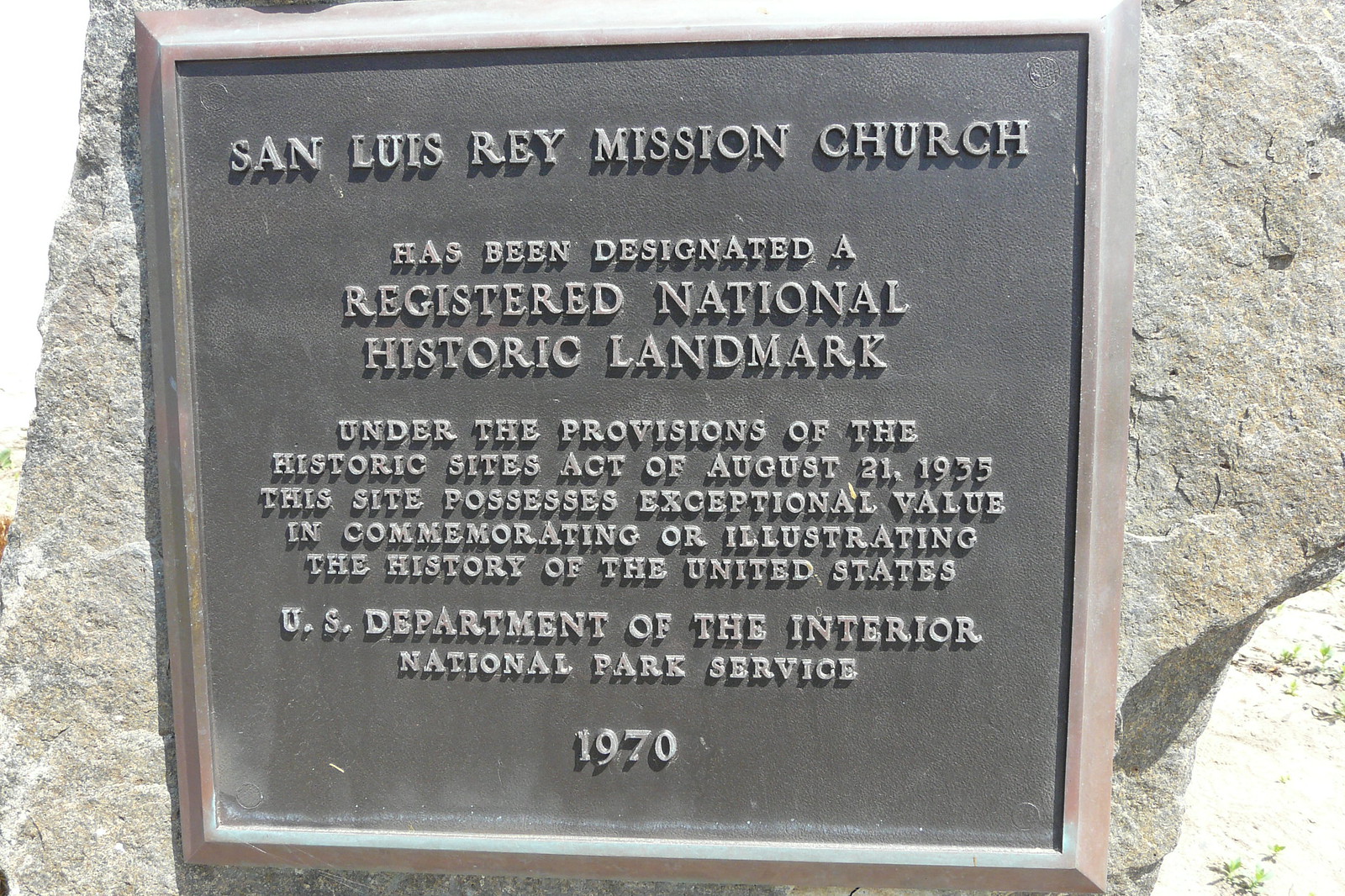The image shows a well-maintained, dark charcoal gray, metal plaque with a slightly lighter gray frame mounted on a rough, gray stone surface. The plaque, featuring raised bronze letters and a bronze border, reads:

"San Luis Ray Mission Church has been designated a registered National Historic Landmark under the provisions of the Historic Sites Act of August 21, 1935. This site possesses exceptional value in commemorating or illustrating the history of the United States. U.S. Department of the Interior, National Park Service, 1970."

The sign, dating back to 1970, designates the San Luis Ray Mission Church as a site of exceptional historical value in the U.S. The plaque is remarkably well-preserved, suggesting regular maintenance.